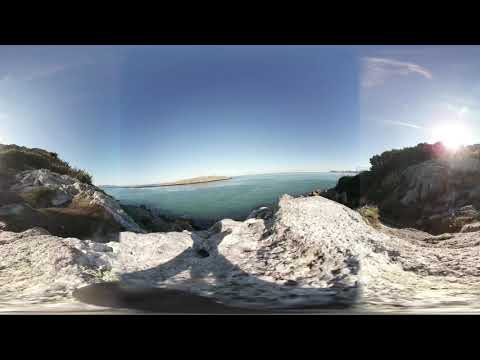In the image, a picturesque bay stretches out before us, characterized by bluish-green waters and a vibrant blue sky dotted with a few wispy clouds. Prominent in the foreground are low knolls of rocks, with patches of grass rising over some of them, creating a natural coastline. On the right, a part of a jetty juts out into the bay, balancing the spit seen extending into the ocean on the left. The water's depth is perceptible through a shift in color, revealing lighter shallow zones near what appears to be a beach on the spit. Additionally, there are formations on the beach resembling large, off-white coral pieces or piled-up sand. In the distance across the water, landmass is visible, perhaps an island, under a serene sky where the faint yellow of the rising sun enhances the scene's tranquil beauty.